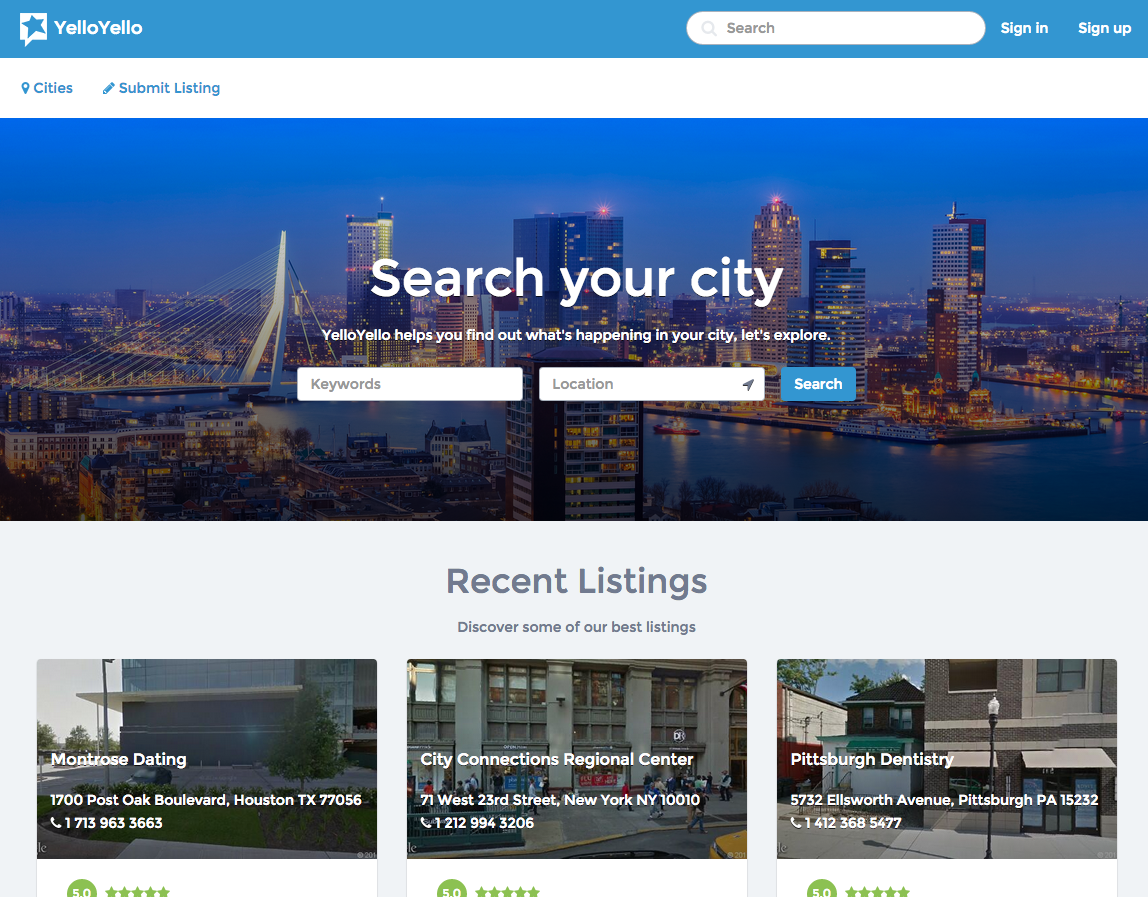A screenshot of a website showcasing a clean and professional design. At the top, there's a sky blue banner with no visible URL. On the left side of the banner, a white text bubble with a blue star contains the phrase "yellow yellow" in white text. On the far right of the banner, there's a white oval search box featuring a grey magnifying glass icon on the left side. To the right of the search box, "Sign In" and "Sign Up" are written in white text.

Beneath the banner, a white space on the left features the blue text links "Cities" and "Submit Listing." Below this section, a banner image displays an aerial view of an industrialized cityscape, potentially representing cities like New York, Chicago, or any other large metropolis. Bold white lettering across the image reads, "Search Your City." Below this, smaller white text states, "yellow yellow helps you find out what's happening in your city. Let's explore."

Underneath the banner image, two white rectangular text boxes are displayed for user input, labeled "Keywords" on the left and "Location" on the right. Next to these, a blue search button with "Search" written in white awaits user interaction.

Further down, on a white background, grey text introduces a section titled "Recent Listings" with the subtitle "Discover some of our best listings." This section features three horizontally aligned images. 

- The first image on the left shows a storefront of a high-rise building labeled "Montrose Dating" located at 1700 Post Oak Boulevard, Houston, Texas. Below it is a green circle accompanied by five green stars.
 
- The central image depicts a bustling business building made of grey stone, labeled "City Connections Regional Center," confirming its New York address. A green dot beneath it indicates a rating of 5.0, shown with five green stars.

- The final listing on the right shows a storefront in an average American downtown area, labeled "Pittsburgh Dentistry" in white text, situated in Pittsburgh, Pennsylvania. Beneath it, a green circle with a white 5.0 and five green stars indicates its rating.